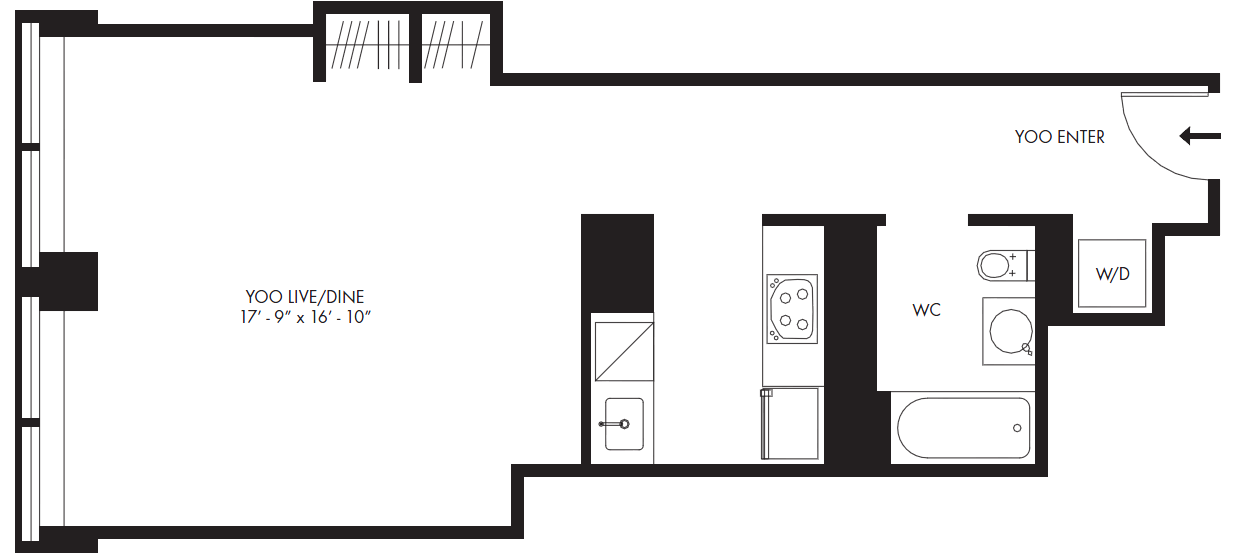This photo layout showcases the blueprints of an apartment, highlighted in white with black outlines demarcating the walls and separating different rooms. The entry point, marked at the top right, is an open doorway with an arrow directing left.

Immediately to the left upon entry, a square space is designated for a washer and dryer unit. Adjacent to this space is the bathroom, which features a bathtub, sink, and toilet.

Continuing past the bathroom, you will find an opening that leads into the kitchen. The kitchen area is equipped with a sink, stove, and refrigerator. 

Proceeding straight from the kitchen, the blueprint opens up into a combined living room and dining room area.

To the right of this combined space, the back wall has a distinctive 'E' shape, oriented sideways. This shape includes several horizontal and vertical lines, adding unique contours to the apartment’s layout.

Additionally, some text within the image reads, "U enter, it's YOO and U live done, it's YOO," which may be a playful or artistic element within the blueprint.